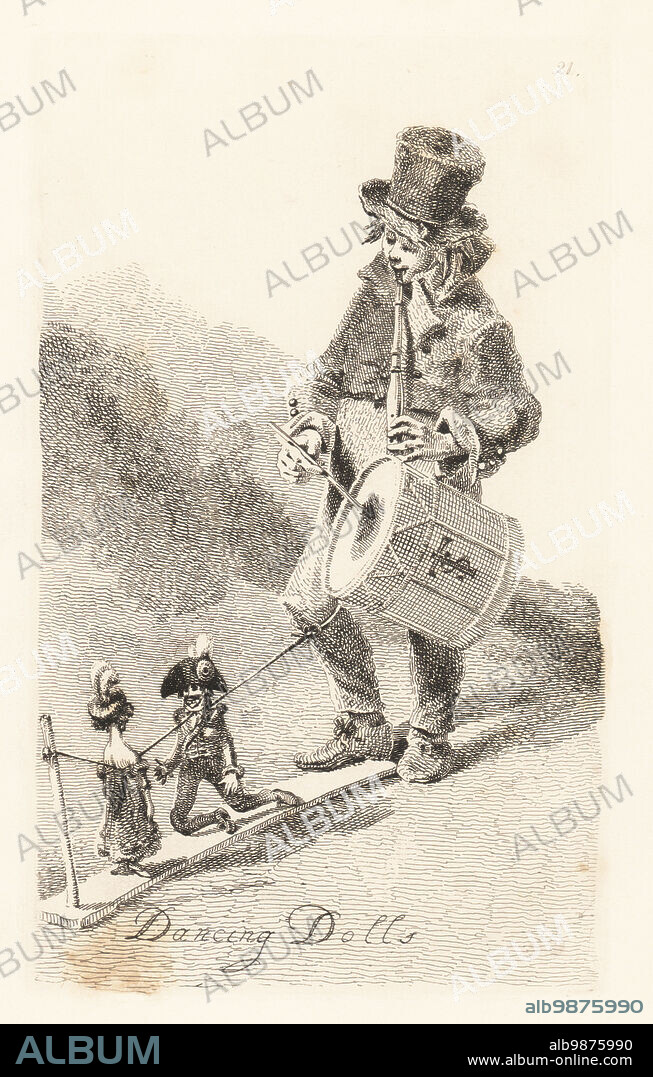The image appears to be a black-and-white sketch or digital graphic depicting a man, possibly a clown or jester, dressed in early 19th-century attire, including a ragged coat, slack shoes, and a top hat. The man is playing a drum and a clarinet-like instrument while manipulating two marionettes attached to strings tied to his leg. The marionettes seem to be dancing or moving as he performs. Overlaid in gray across the entire image, the word "ALBUM" is repeatedly printed, likely as a form of copyright protection. Below the illustration in a cursive script, the title "Dancing Dolls" is written. Further down, on a black banner, there is text that reads "ALBUM" along with the identifier "ALB9875990" and the web address "www.album-online.com," indicating the source of the image. This appears to be a preview of an image available for purchase or download.